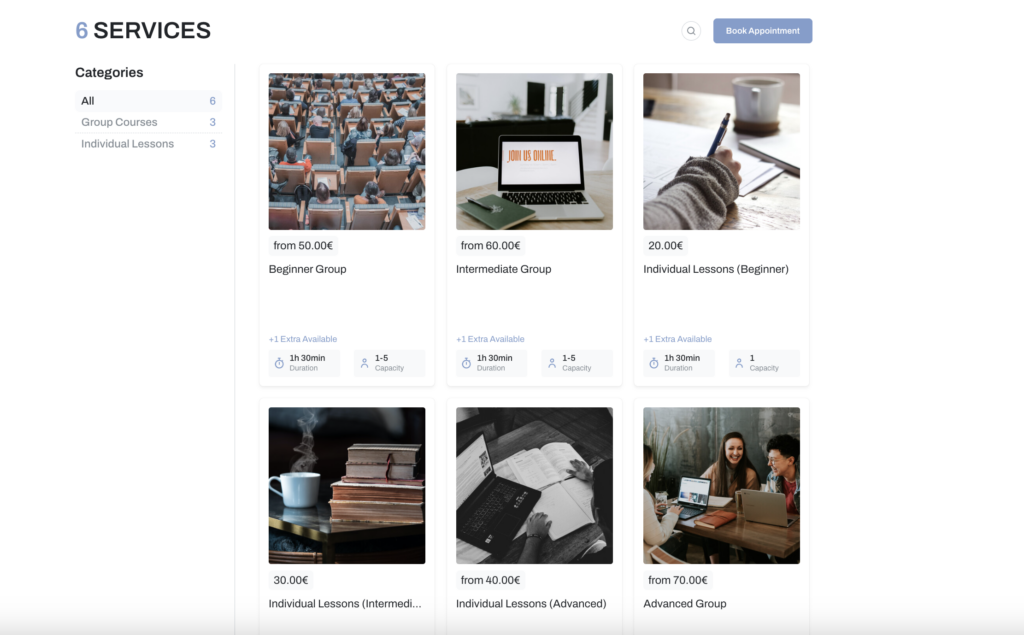On a service-oriented website, the top-left corner prominently displays a gray number "6", next to the word "services" in bold black font, indicating the availability of six distinct services. Adjacent to this, a small magnifying glass icon encased in a light blue circle offers a search functionality for navigating through these services.

To the far right of the same top bar, a notable blue rectangular button with "Book Appointment" inscribed in white font invites users to schedule appointments for their chosen services. Directly beneath the "6 services" label, a "Categories" section appears in black font. It segments the services into three distinct groups: "All," "Courses," and "Individual Lessons."

Within the "Courses" category, users can explore six different offerings, each accompanied by a small thumbnail image and varying price points. The courses are further classified into "Beginner Group," "Intermediate Group," and "Individual Lessons for Beginners." Each section provides a detailed and visual guide to help users select the appropriate learning path tailored to their needs.